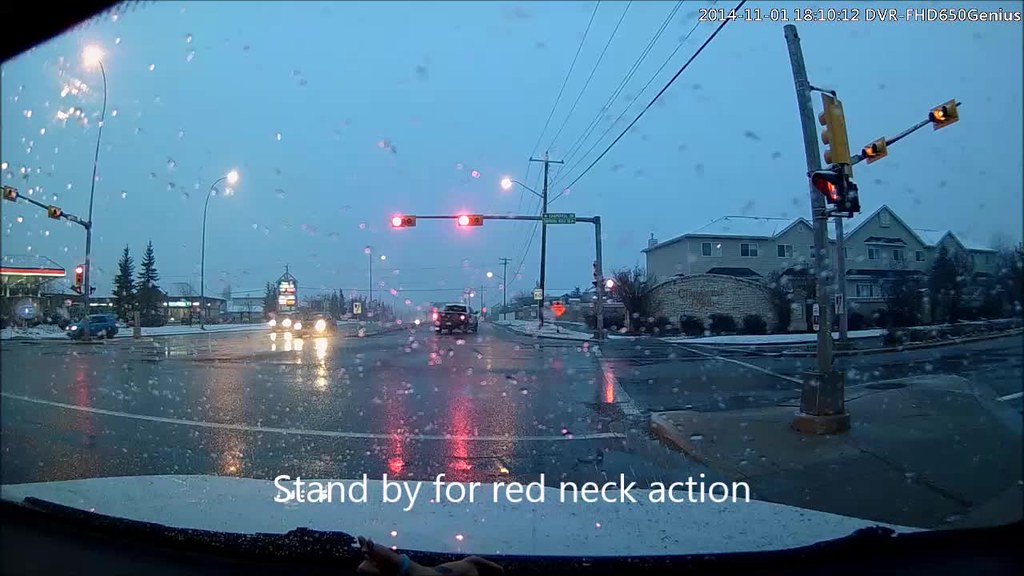This photograph captures a bustling, expansive intersection on a dreary day, with a mix of rain and light snow falling from the cloudy sky. Central to the image is a large condominium complex dominating one corner of the intersection, while a gas station occupies the opposite corner. The road itself is notably wide, hinting at its significance in the area's traffic flow.

Further down the street, a series of various stores line the road, their signs barely visible through the precipitation. The ground has a light dusting of white, remnants of the early snowfall mixed with rain.

A truck has just moved through the intersection, leaving behind a scene of anticipation as various vehicles wait to navigate through. Among these, two cars face straight ahead, poised to continue on their path, while another car is positioned to make a right turn.

The perspective suggests the photograph was taken from within a vehicle, evident by the hint of the dashboard and part of the windshield framing the scene. A caption accompanying the image reads, "Stand by for redneck action," possibly hinting at the imminent negligence of traffic rules – specifically the anticipation of a driver attempting to run the yellow light, risking it turning red.